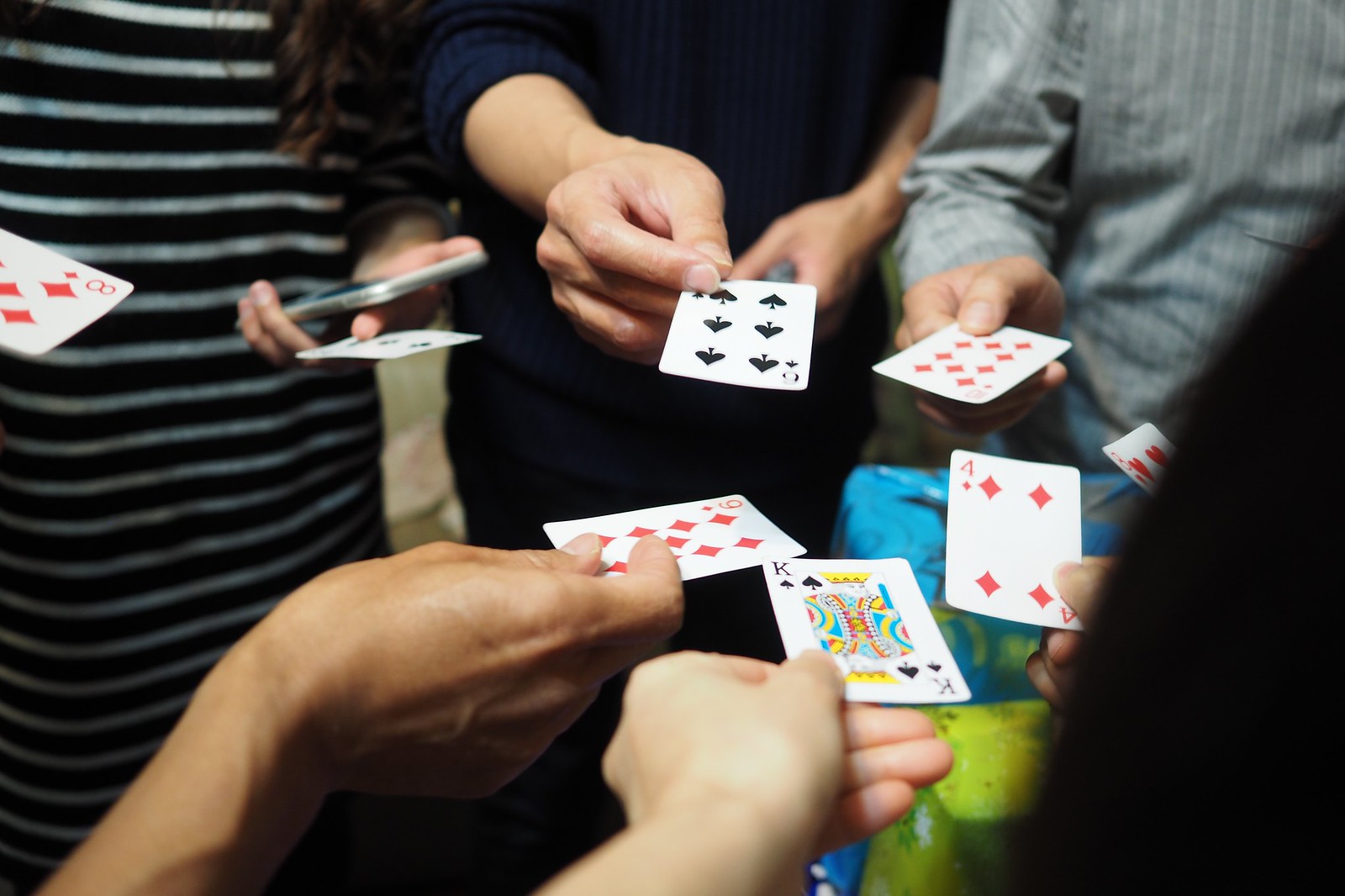A vivid photograph captures five individuals deeply engaged in a card game. The scene centers around a circular arrangement of players, each attentively holding a card in each hand towards the center of the circle. One player, dressed in a black outfit adorned with white horizontal stripes, contrasts sharply against another participant clad in a gray long-sleeved shirt, featuring blue and gray vertical stripes. Although the face of one player is obscured, their presence is felt through a pair of hands gripping a set of cards. Key cards visible include the eight of diamonds, nine of diamonds, six of spades, and four of diamonds, highlighted by the well-illuminated setup. The blurred back of a black-haired individual's head in the foreground adds a layer of depth to the image. The green and blue hues in the backdrop, possibly indicative of a table, suggest where the game unfolds. This close-cropped image focuses on the players and their cards, leaving the surrounding environment a mystery.